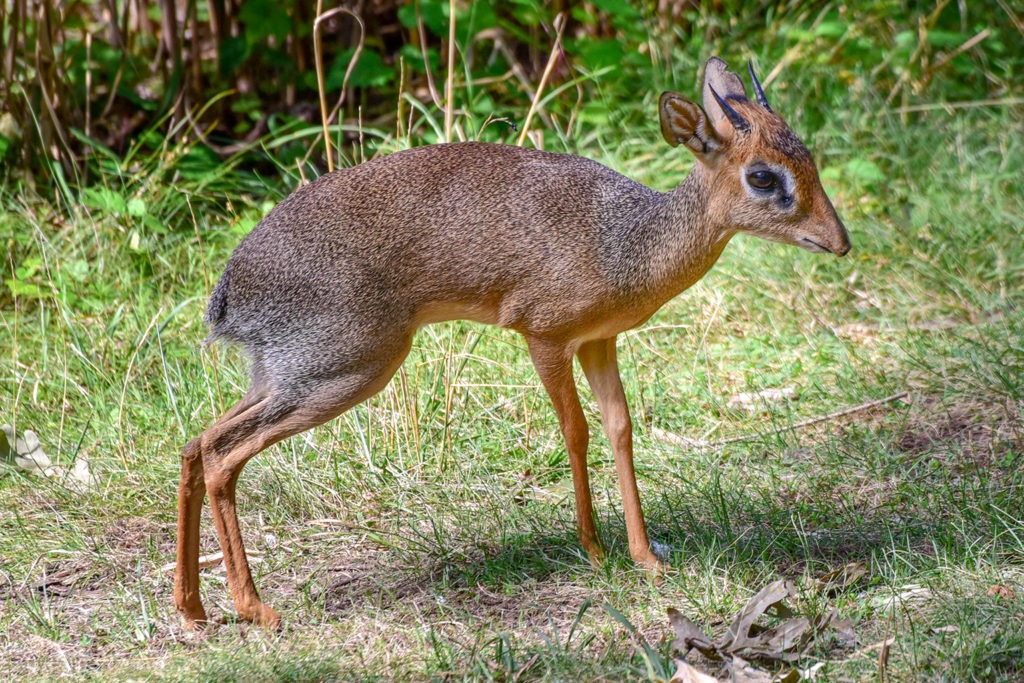In this vibrant nature photograph taken on a sunny day, a young, brown antelope-like animal, possibly mistaken for a deer, stands cautiously in a grassy area filled with a mix of green and brown patches. The animal, with small budding horns suggesting it's a male, has an alert and somewhat scared expression, its legs slightly crossed as if it has just stood up for the first time. Its fur is primarily brown with specks of gray, black, and white, adding to its unique appearance. The background is lush with greenery, featuring various foliage, small trees, vines, and a few scattered sticks and dead leaves, creating a rich and natural forest-like setting. The baby animal looks directly at the camera, set against the vivid natural backdrop, forming a harmonious blend of innocence and wild beauty.